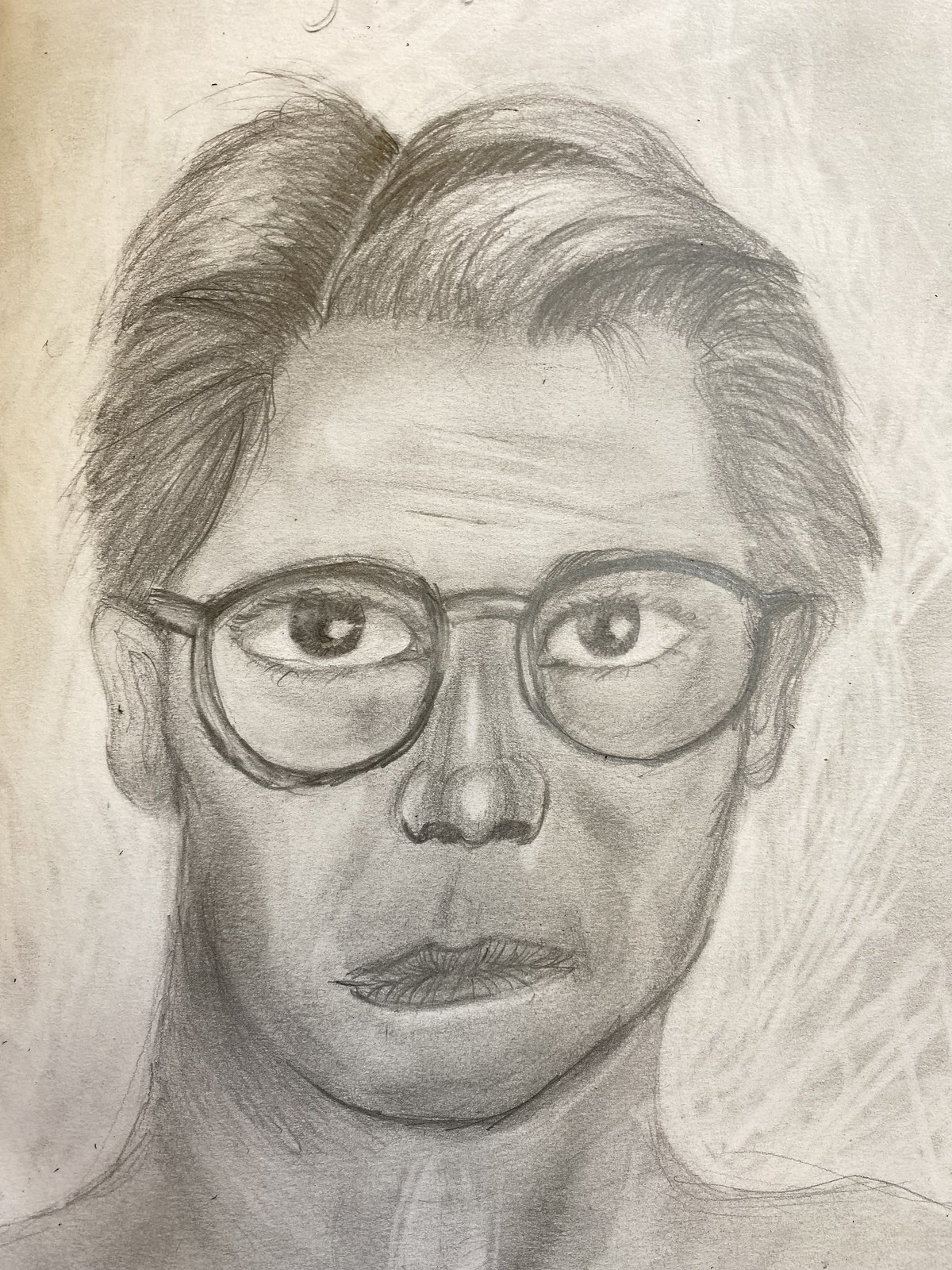This is a photograph of a detailed pencil sketch of a man in his mid-30s to mid-40s, depicted from the shoulders up. The image is drawn entirely in black and white. The man has short, dark hair, which is combed and parted to his right side, appearing slightly overgrown. He wears circular, black-framed glasses, though the frames are asymmetrical with the left side being slightly larger. His large, almond-shaped eyes, one being darker and both open wide, are not symmetrically shaped, adding to the slightly unrefined quality of the illustration.

Despite the detailed shading and effort, the man's facial features appear somewhat poorly executed, resulting in an unnatural look. His forehead has visible wrinkles, and he sports a small, rounded nose with detailed shading. His thin lips are slightly crooked, with the right corner tilting upwards. The sketch reveals a long, flat philtrum above his lips.

The man's ears are small, almost resembling butterfly wings, lacking significant detail. His jaw is square but asymmetrical, leading down to a thick neck and narrow shoulders, giving the impression that he might not be wearing a shirt. Notably, the shading in the image is darker on the left side than on the right, and there's an absence of any background or text. The hair is the most refined part of the sketch, with each strand meticulously detailed, contrasting with the underwhelming quality of the facial features.